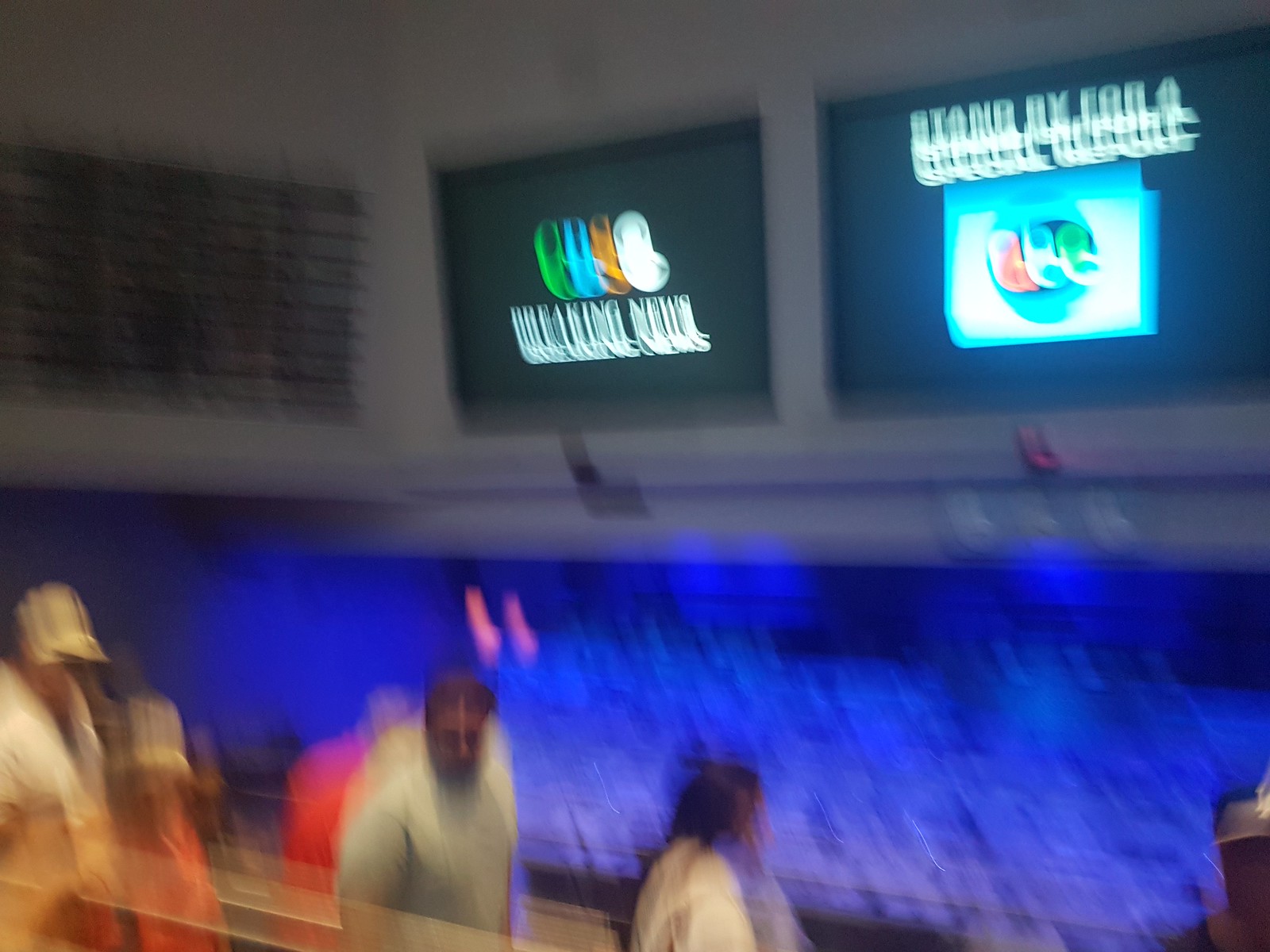In this indoor, blurry photograph, the top half showcases a white wall adorned with two television screens, each displaying extremely indistinct images. The screen on the left appears to feature the logo for CBS, while the one on the right seems to show ABC. Adjacent to these screens, on the left side of the wall, is a black rectangle. The lower section of the photograph is dominated by a blurred, mixed-color backdrop primarily composed of purple, white, and black hues. At the very bottom of the image, several indistinct figures can be observed. On the left edge is the right profile of a person donning a white cap and a white top. Next to this individual stands a shorter person clad in an orange outfit with a white hat. To their right, a man with dark hair, slightly bent over, is seen wearing a white t-shirt. Faces and other finer details are indistinguishable due to the blur.